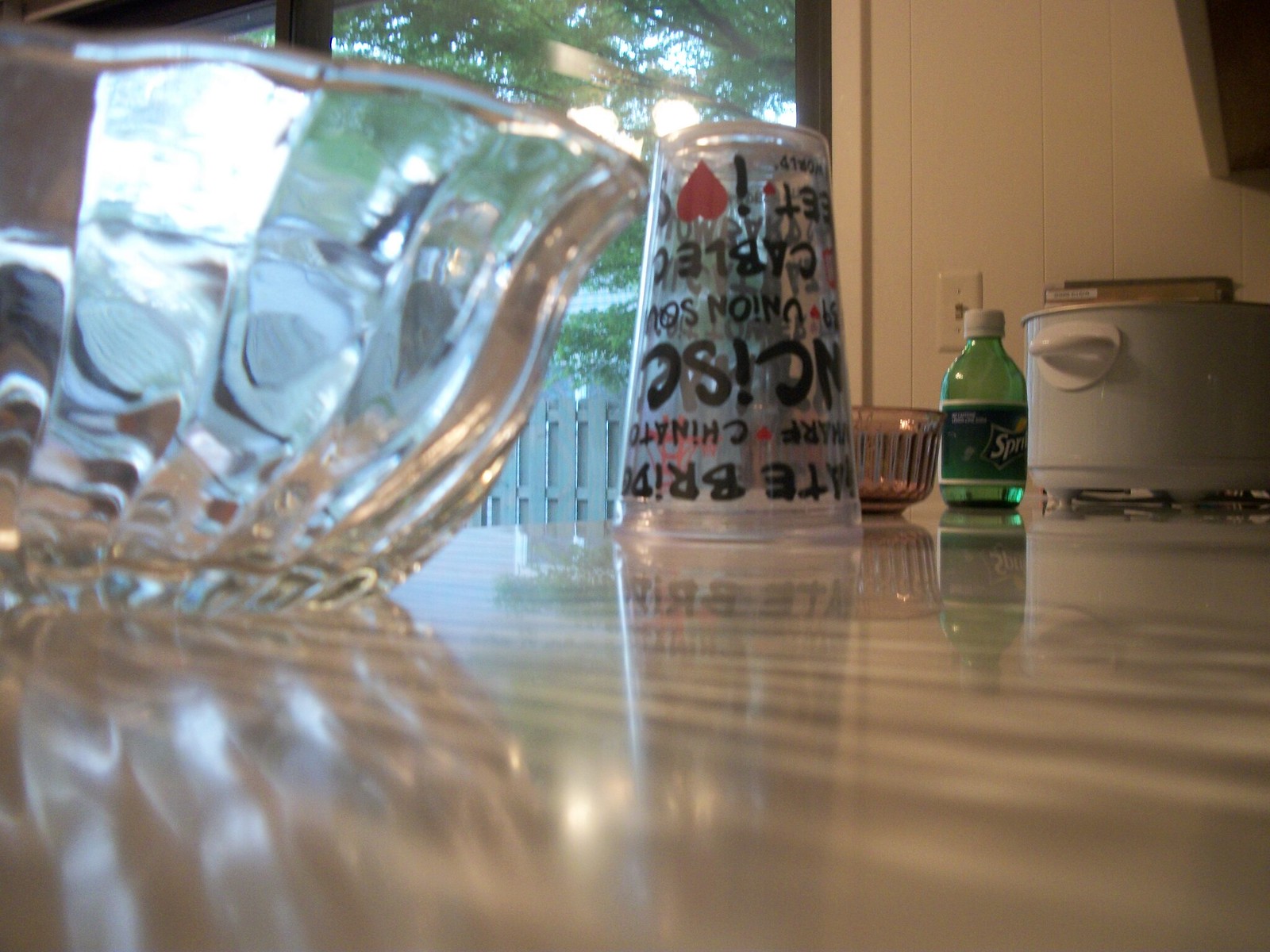This photograph appears to have been taken from a vantage point right on top of a table, capturing a detailed scene both on the table and beyond it. On the left side of the table, there is a large, scalloped glass bowl. Directly ahead on the table, there is a plastic cup featuring black text on its surface. Behind this cup sits a shorter, scalloped pink glass bowl. Next to it and slightly behind is a stubby, short glass spray bottle. To the right of the spray bottle is a white crock pot. In the background, a white wall with a white light switch can be seen. Looking beyond the table, the view extends outside to reveal a gray fence, a tree, and a patch of sky.